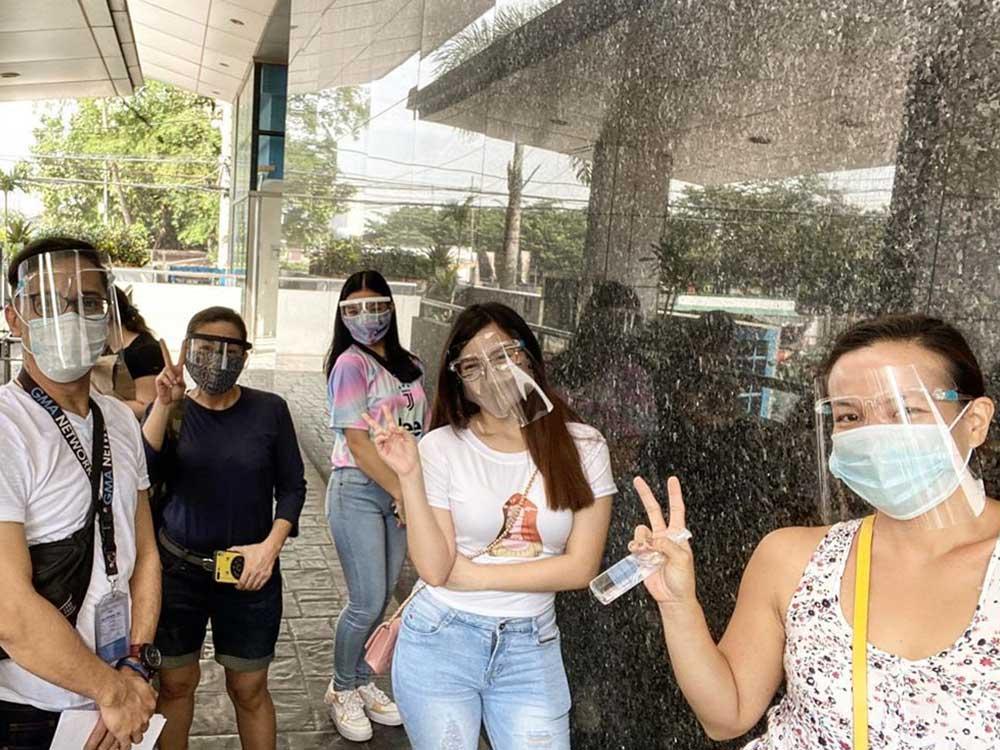The photograph captures a group of people, likely taken recently during the COVID-19 pandemic. All individuals are wearing both white paper masks over their mouth and nose, as well as clear face shields, reflecting the health precautions of the period. The image includes three young women who are all posing with peace signs and a man who has a badge around his neck, possibly indicating entry to some event or convention. The man stands with his arms in front of him, folded at his side. 

The scene is set outside a building that features highly reflective, mirror-like walls, doubling the visuals in the surrounding area and creating an impression of water or a shower-like feature in the background. This reflective wall is likely made of a modern, smooth material like glass or marble. The environment also includes trees and sky visible through the glass walls, suggesting the building has transparent walls to blend the interior with the exterior. The flooring appears to be concrete.

Everyone in the photograph appears to be of Asian descent, with dark hair and relatively young appearances, dressed casually in jeans and short white shirts. The harmonious yet strict adherence to COVID-19 preventative measures and their shared fashion sense create a unified and contemporary image of life during the pandemic.